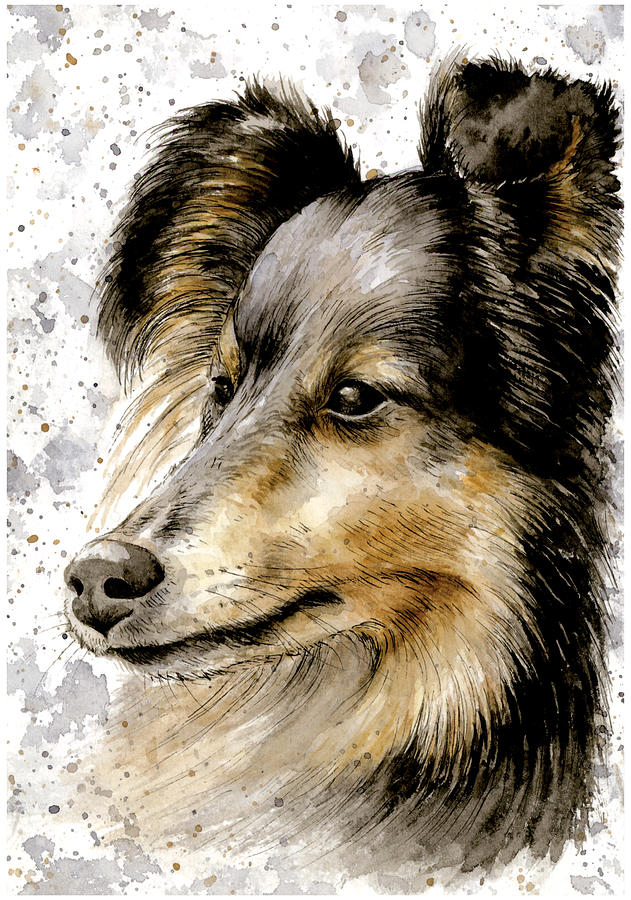This image is a detailed painting of a border collie, focusing on its face from the neck up. The dog's side profile is directed towards the left, showcasing its long nose and well-perked, fluffy black ears which have white stripes running down them. The dog's forehead features a dark grayish-black coloration, while its cheeks and the area under its chin display white and tan shades, intertwined with brownish-yellow patches. The eyes are black with a slight shine or reflection, adding a touch of realism. Whiskers are also visible on its face, enhancing the intricate detail. The background is an abstract mix of colors, primarily white with splashes and dots of red, blue, brown, rust, and gray scattered in a random pattern, lending a vibrant yet artistic backdrop to the composition.